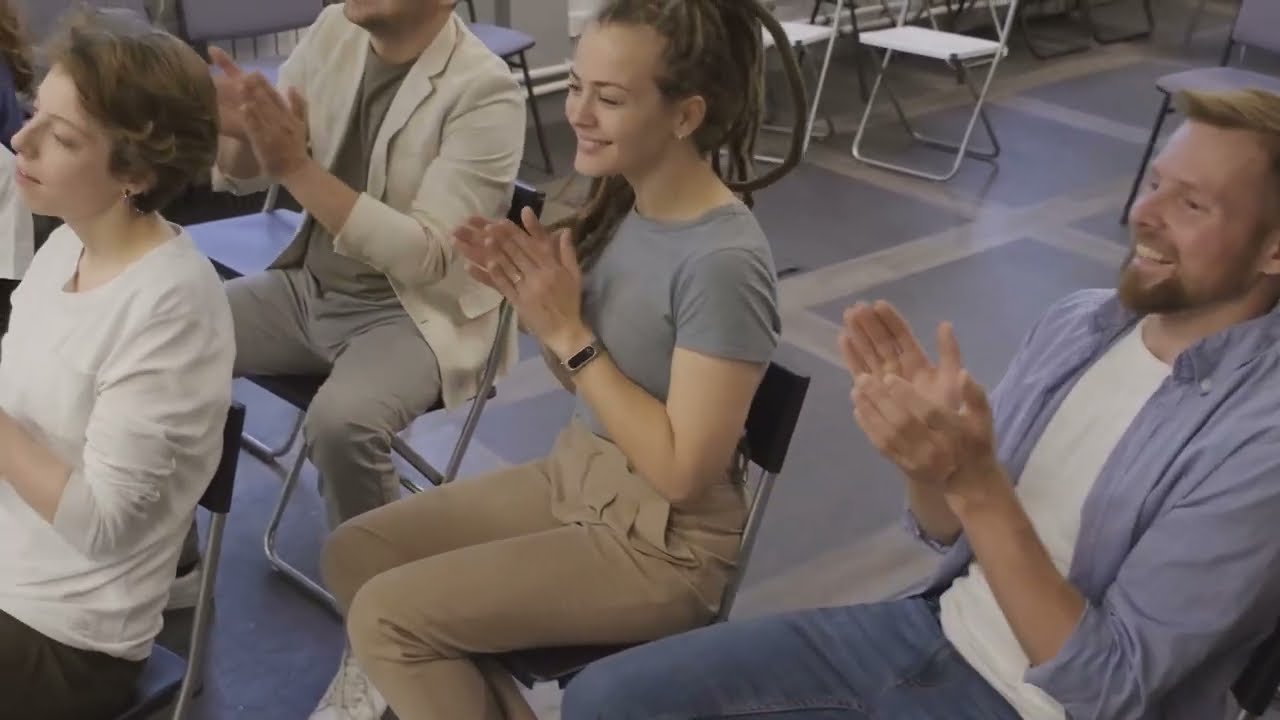The image depicts a room with a tiled floor featuring large gray squares and smaller paths in between. Several people are seated on folding chairs arranged in rows, with additional empty chairs visible in the background. The individuals are all clapping and looking forward, appearing to be watching something. 

On the right side of the image, there's a man with short blondish-brown hair, a beard, and a mustache. He is wearing a white t-shirt under an unbuttoned blue collared long-sleeve shirt with rolled-up sleeves, along with blue jeans. Next to him, centrally positioned, is a smiling woman with long brown hair styled in tight braids, dressed in a short-sleeve gray t-shirt and brown pants, also wearing a Fitbit on her left wrist.

To her side is another man dressed in a light beige suit jacket with a brown t-shirt underneath and gray pants, although his head is cut off by the top edge of the photo. Additionally, there is a woman in the foreground on the left with short brown hair, wearing a long-sleeve white shirt with the sleeves pulled back and dark slacks. Everyone in the image is smiling and appears to be engaged in the activity.